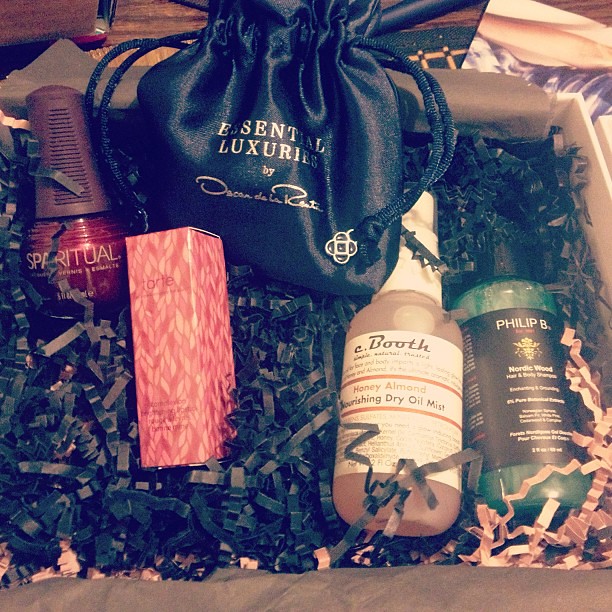This close-up image showcases a meticulously arranged gift box filled with beauty products nestled in dark, frilly, crinkled confetti-like paper. At the forefront on the right is a green bottle with a black label reading "Phillip B. Nordic Wood Hair and Body Shampoo." To the left of this bottle is another container labeled "Booth Honey Almond Nourishing Dry Oil Mist," featuring a white label. Above these products, there's a sophisticated black drawstring bag labeled "Essential Luxuries." Beneath this bag lies a rectangular pink box inscribed with the brand name "Tarte." Additionally, towards the upper left side of the box, there's a distinctive bottle labeled "Spiritual," containing a striking red substance, likely nail polish. The entire ensemble is presented against a wooden table background, exuding an aura of luxury and careful curation ideal for beauty enthusiasts.